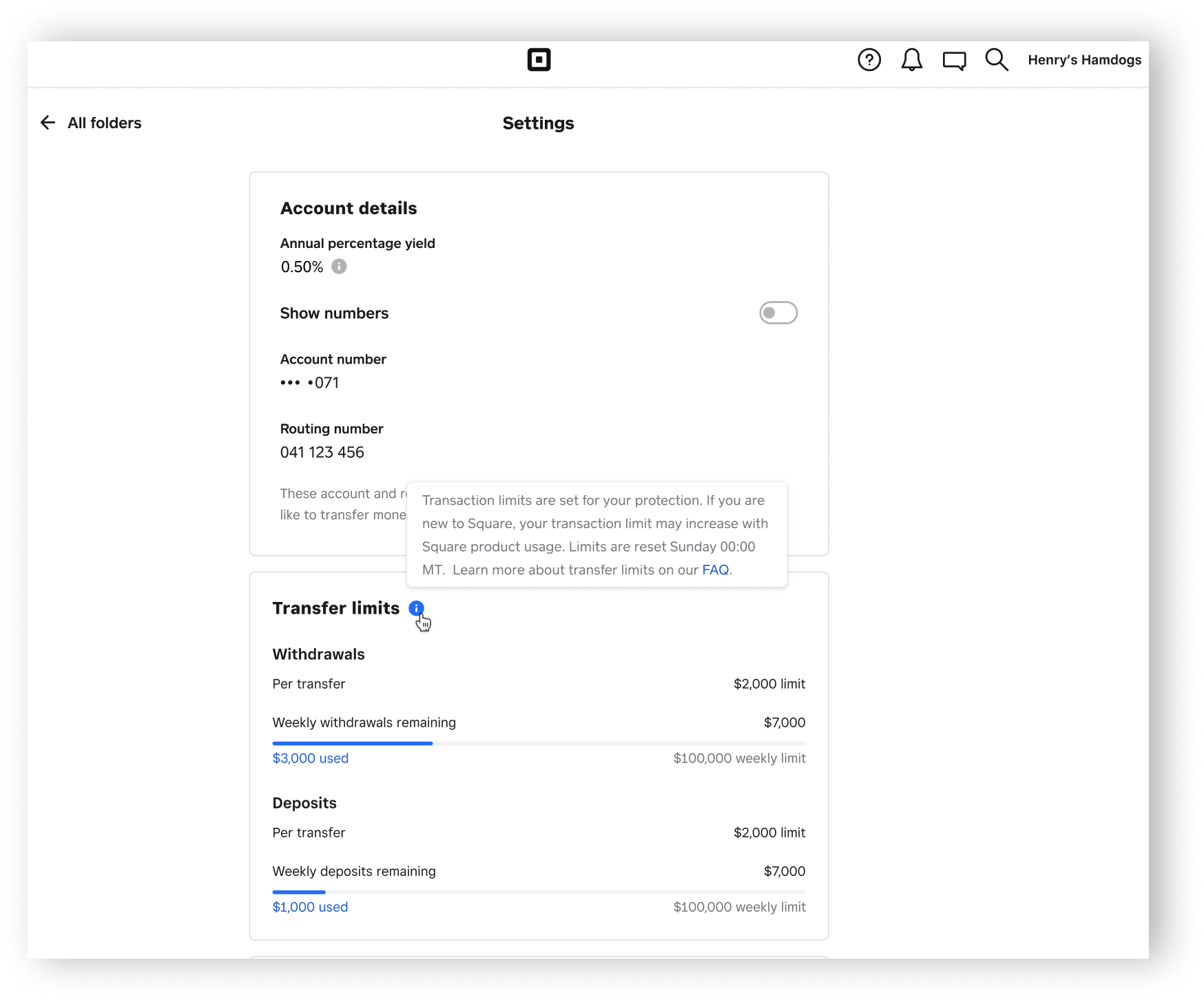The image is a horizontally rectangular screenshot with a white background, indicating it's likely from an app or website. The upper-right corner prominently features the text "Henry's Ham Dogs," suggesting the brand or platform in question. Centrally placed in bold black font is the heading "Settings." Directly underneath, two boxes outlined in a very thin light gray contain detailed information.

The top box focuses on account specifics with the following details:
- **Account Details**
  - **Annual Percentage Yield**: 0.50%
  - **Account Number**: Partially obscured by asterisks with only the last three digits visible as "071."
  - **Routing Number**: 041123456
  Additionally, there is a toggle button next to the Annual Percentage Yield information, which is currently set to off.

Covering part of the information below the Routing Number is a pop-up window associated with the second box titled "Transfer Limits." The mouse hand cursor is seen clicking on an information ("i") button, triggering the pop-up window which reads:
- **Transaction limits are set for your protection. If you are new to Square, your transaction limit may increase with usage of Square products. Limits are reset every Sunday at 00:00 Mountain Time. Learn more about Transfer Limits on our FAQ** (where "FAQ" is a clickable blue link).

The precise layout and interactive elements indicate the functionality and user interface design of the platform.